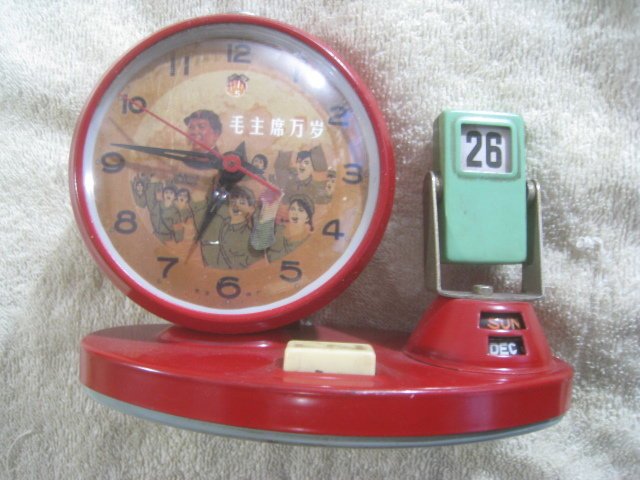This photograph features a vintage-style red metal clock set against a white carpet background. The clock appears to have Chinese influences, suggested by both the Asian figure and characters present on its face. The clock is designed with a dual display, showcasing the time and date. It reads 7:46, with black hour and minute hands, and a red second hand standing out against its dark brown face. The date section prominently displays "Sunday, December 26" with "S.U.N." for Sunday above it. Notably, the date indicator features a green, gas tank-shaped area with the number 26 in black. This retro clock, with its unique design elements, reflects a blend of functionality and cultural aesthetics.